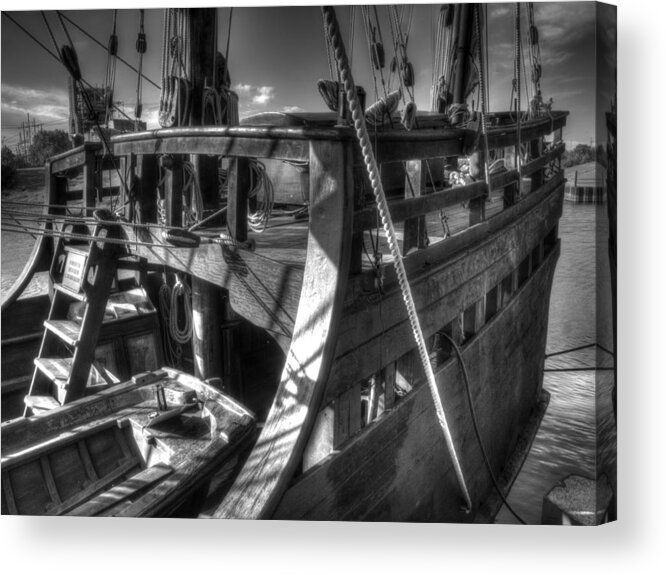This black-and-white photograph vividly captures an old-time wooden ship moored in the water, its image framed in a sturdy border that is a few inches thick, adding a sense of depth. The vessel, larger than a typical speedboat but not overwhelmingly huge, is adorned with a myriad of ropes and sail pulleys, indicative of its sailing purpose. A ladder extends to the upper deck, hinting at a vessel substantial enough for someone to sleep on. The ship is tied to what appears to be a dock, with the tethering rope prominently visible at the front. The scene is bathed in light, likely from moonlight or a large spotlight, enhancing the ship's details against a clear sky dotted with a few clouds. An unreadable sign is also present, adding an element of mystery to the historical ambiance.